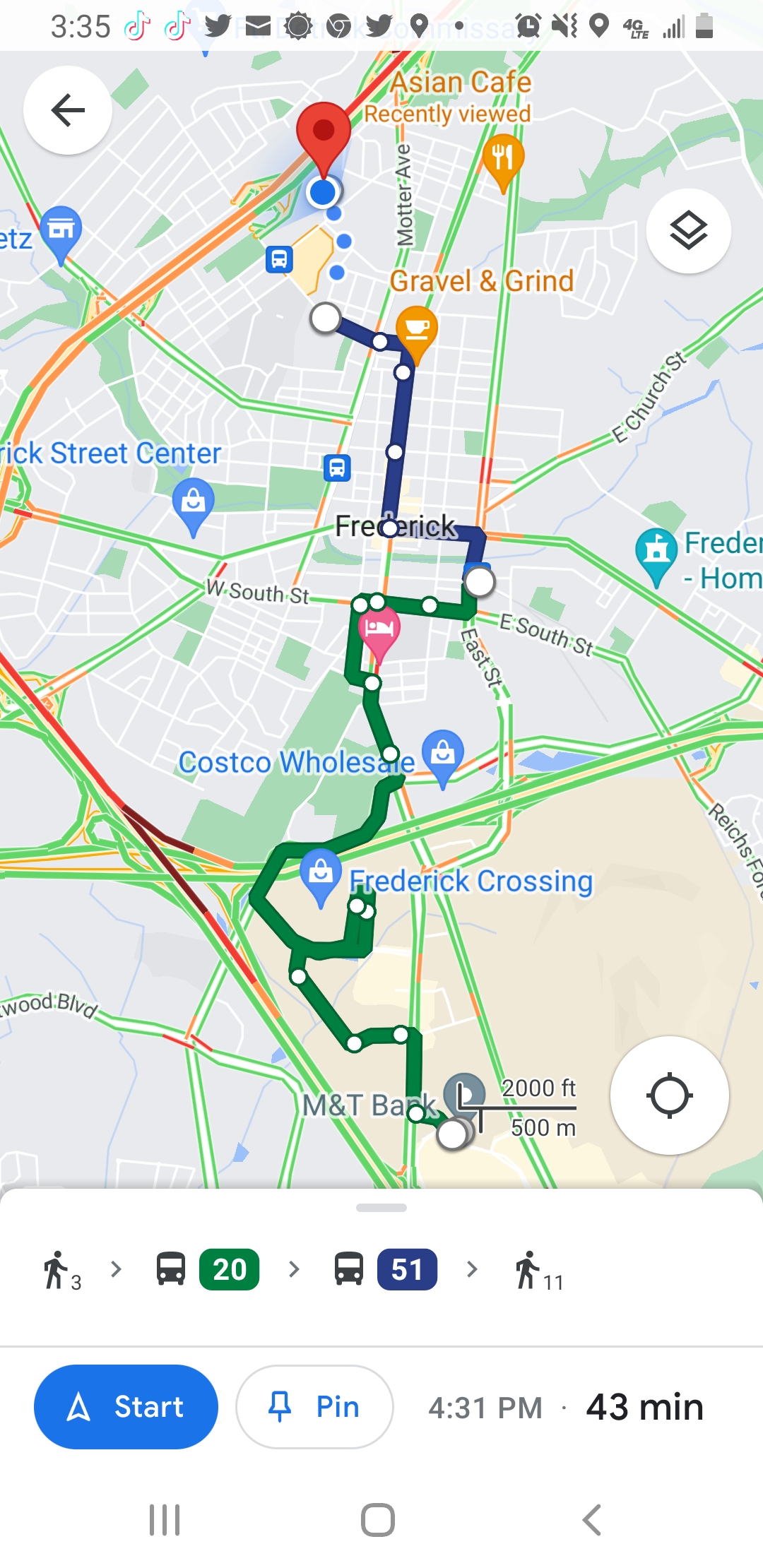This image is a detailed screenshot from a smartphone displaying navigational directions on Google Maps. At the top of the screenshot, various smartphone interface icons are visible, including those for Twitter, TikTok, a digital clock showing the current time, and an alarm notification. The directions depicted are for a route from the southern part of a town to its northern section. The map highlights different transit steps, starting with a pedestrian icon, indicating a walking segment. This is followed by symbols for two bus routes, the 20 and 51, suggesting transfers between buses. The navigation route concludes with another walking symbol, illustrating the final leg of the journey.